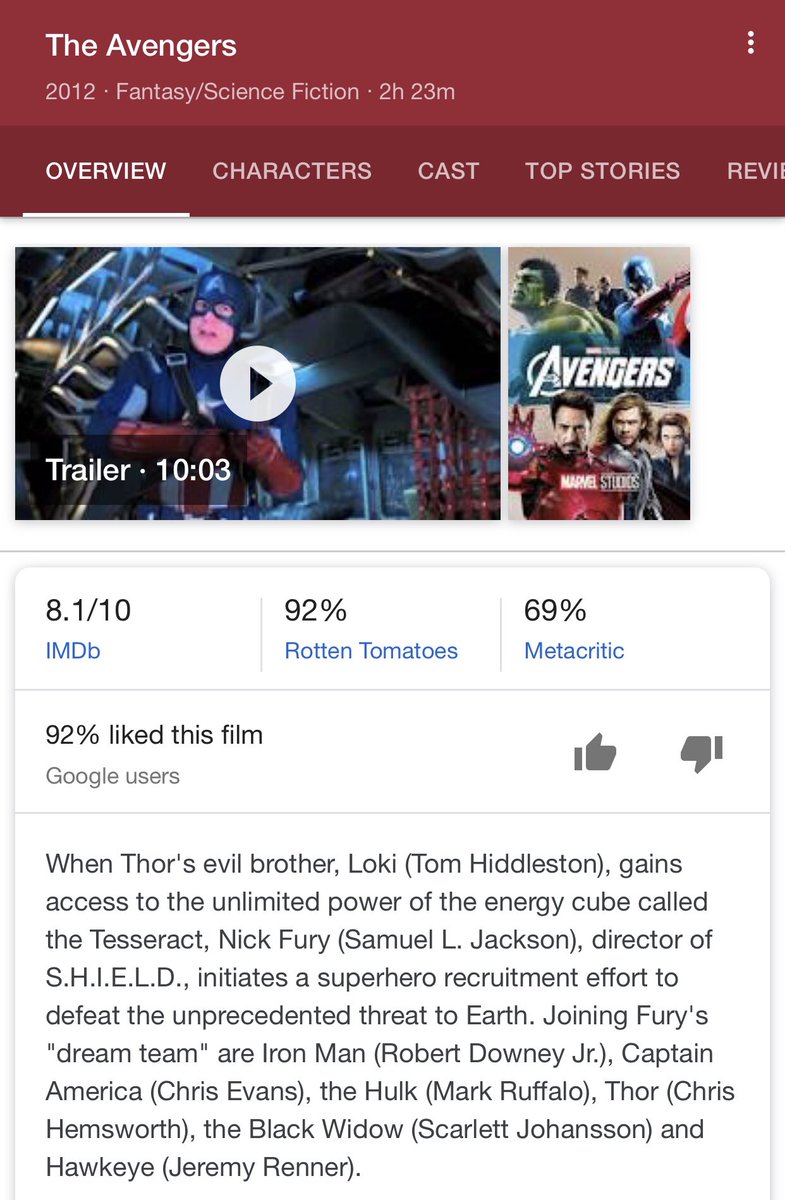This image is a detailed screenshot of the Rotten Tomatoes page for the movie "The Avengers" (2012). The header is a light burgundy color with "The Avengers" in white text, followed by "2012, Fantasy/Science Fiction, 2 hours 23 minutes" in light pink. Below the header is a darker burgundy menu bar featuring options such as "Overview," "Characters," "Cast," "Top Stories," and "Reviews," with "Overview" underlined.

On the left side of the screen, there's a still frame from the movie trailer that lasts 10 minutes and 3 seconds. The frame features Captain America, with a video play button overlay. On the right side, there's a movie poster showing various Avengers characters, with "Marvel Studios" at the bottom.

The ratings displayed show an 8.1/10 from IMDb, 92% on Rotten Tomatoes, and 69% on Metacritic. There are also up and down thumbs for user voting.

The synopsis highlights the plot: When Thor’s evil brother Loki (Tom Hiddleston) gains access to the unlimited power of an energy cube called the Tesseract, Nick Fury (Samuel L. Jackson), Director of S.H.I.E.L.D., initiates a superhero recruitment effort to combat the unprecedented threat to Earth. The team includes Iron Man (Robert Downey Jr.), Captain America (Chris Evans), Hulk (Mark Ruffalo), Thor (Chris Hemsworth), Black Widow (Scarlett Johansson), and Hawkeye (Jeremy Renner).